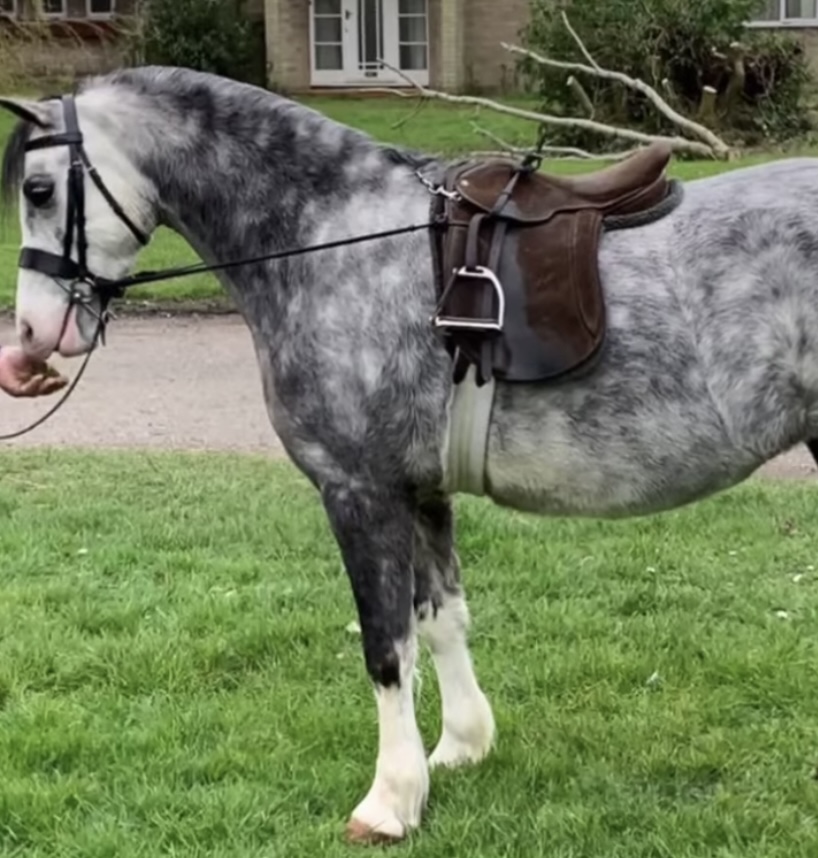This detailed color photograph features a dappled gray horse with black and white marbled fur. The horse, wearing a brown leather saddle secured with straps under its belly, has a white face with smoky-colored eyes and a black forelock. It stands on short green grass, facing left, and tilting its head down to accept something from a partially visible human hand, likely offering it food. Only the front legs of the horse are visible, which are white, contrasting with the rest of its light gray body speckled with patches. In the background, a path runs horizontally with green shrubbery nearby, leading to a barely visible house with part of a door peeking through, along with a tree. The horse's mane is brushed to the side opposite the viewer.